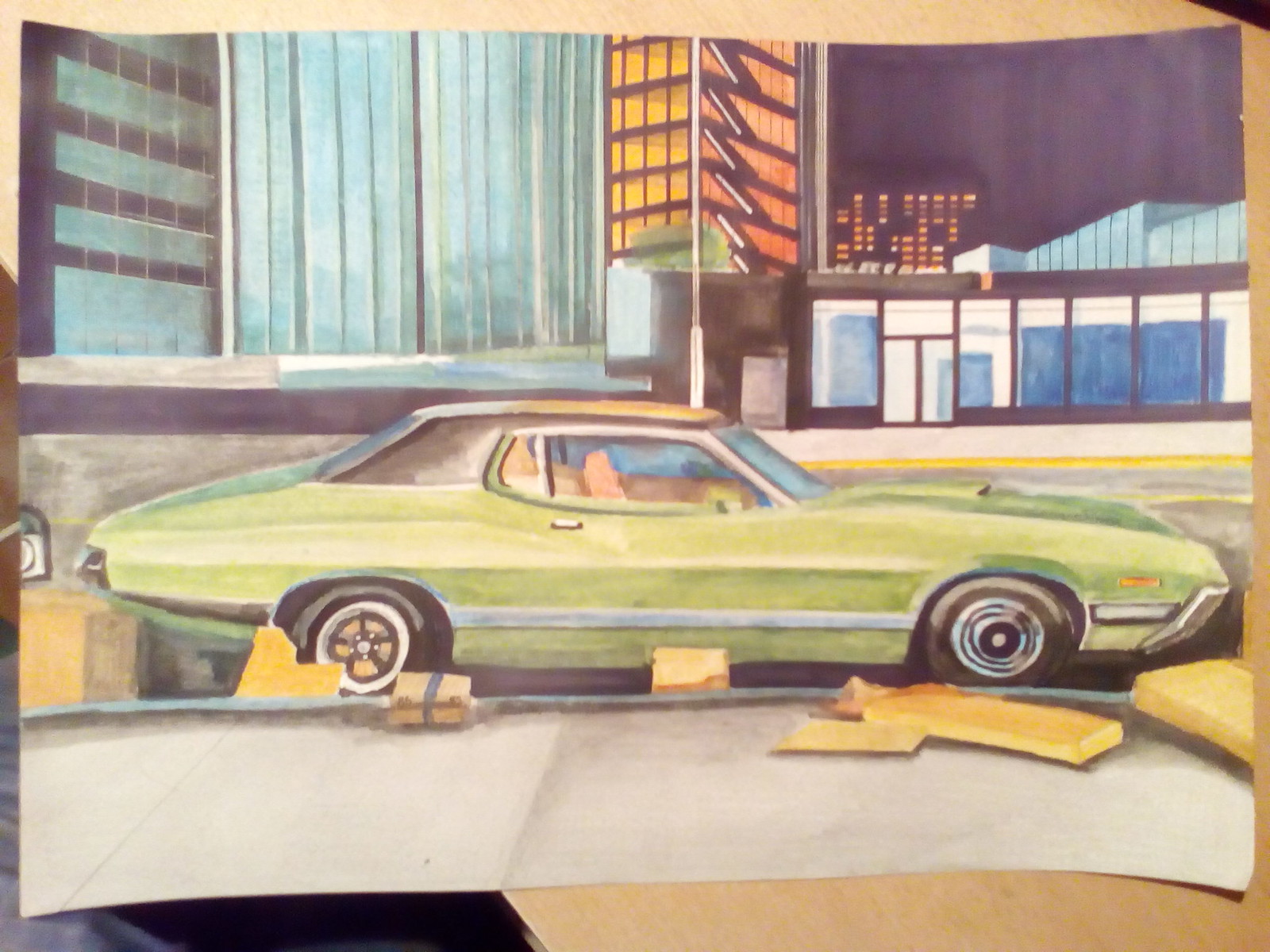The image depicts a large piece of paper adorned with either a painting or a meticulous coloring that centers around a classic muscle car, viewed from the side in a vivid light green hue. The car, a sleek two-door model with a compact backseat, boasts strikingly blue windows and black tires that shine with a noticeable glare. Set against a backdrop of a modern cityscape, the illustration features an array of glass skyscrapers in various hues: turquoise on the left, orange and yellow in the middle, and a mix of black, blue, and yellow on the right. Below, the scene includes a standard traffic street with the car seemingly parked at the edge near a curve. The sidewalk beneath it is rendered in a light gray shade, completing the urban tableau.